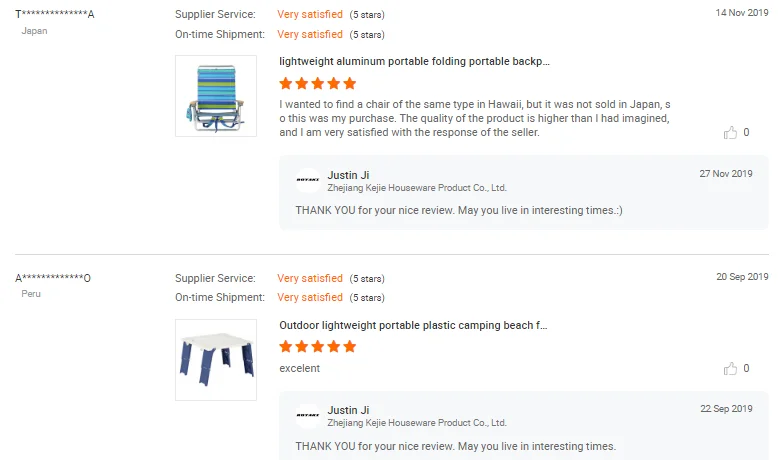**Detailed Product Comparison Review: Lounger vs. Camping Chair**

**Image Description:**
The image showcases a detailed comparison between two different portable seating products: a lightweight aluminum folding lounger and a portable plastic camping chair with legs. Each item's features and customer reviews are presented.

**1. Aluminum Folding Lounger:**
- **Visual Description:** The lounger is primarily striped in blue and green, and includes supportive straps underneath. It is highlighted on the left side of the image.
- **Specifications:** Lightweight, made of aluminum, and portable with a folding design. It's suggested to be a suitable option for backpacking.
- **Customer Review Details:**
  - **Review Date:** November 14, 2019
  - **Customer Satisfaction:**
    - Supplier service: Very satisfied (five stars, orange)
    - Longtime shipment: Very satisfied (five stars, orange)
  - *Review Comment:* The reviewer expresses satisfaction with the product's quality, exceeding their expectations. They mention a desire to find a similar chair in Hawaii, noting that it's not sold in Japan.
  - **Company Response:** On November 27, 2019, a representative named Justin responded, thanking the customer for their positive review and adding a peculiar remark about living in interesting times.

**2. Plastic Camping Chair:**
- **Visual Description:** This chair is white with legs, clearly designed for outdoor use. Positioned on the right side of the image.
- **Specifications:** Lightweight, foldable, and made of durable plastic, ideal for camping or beach settings.
- **Customer Review Details:**
  - **Review Date:** September 20, 2019
  - **Customer Satisfaction:**
    - Water service: Very satisfied
    - On-time shipping: Very satisfied (both ratings in orange)
  - *Review Comment:* The reviewer, anonymized with a name ending in "0" or "O" and apparently from Peru, comments positively on the product's excellent condition.
  - **Company Response:** Similar to the response for the lounger, the reviewer received a thanks for their nice review with the same enigmatic comment about living in interesting times. This interaction occurred two days after the initial review.

Overall, both products received high satisfaction ratings from the reviewers, with the company acknowledging each review with appreciative and peculiar remarks.